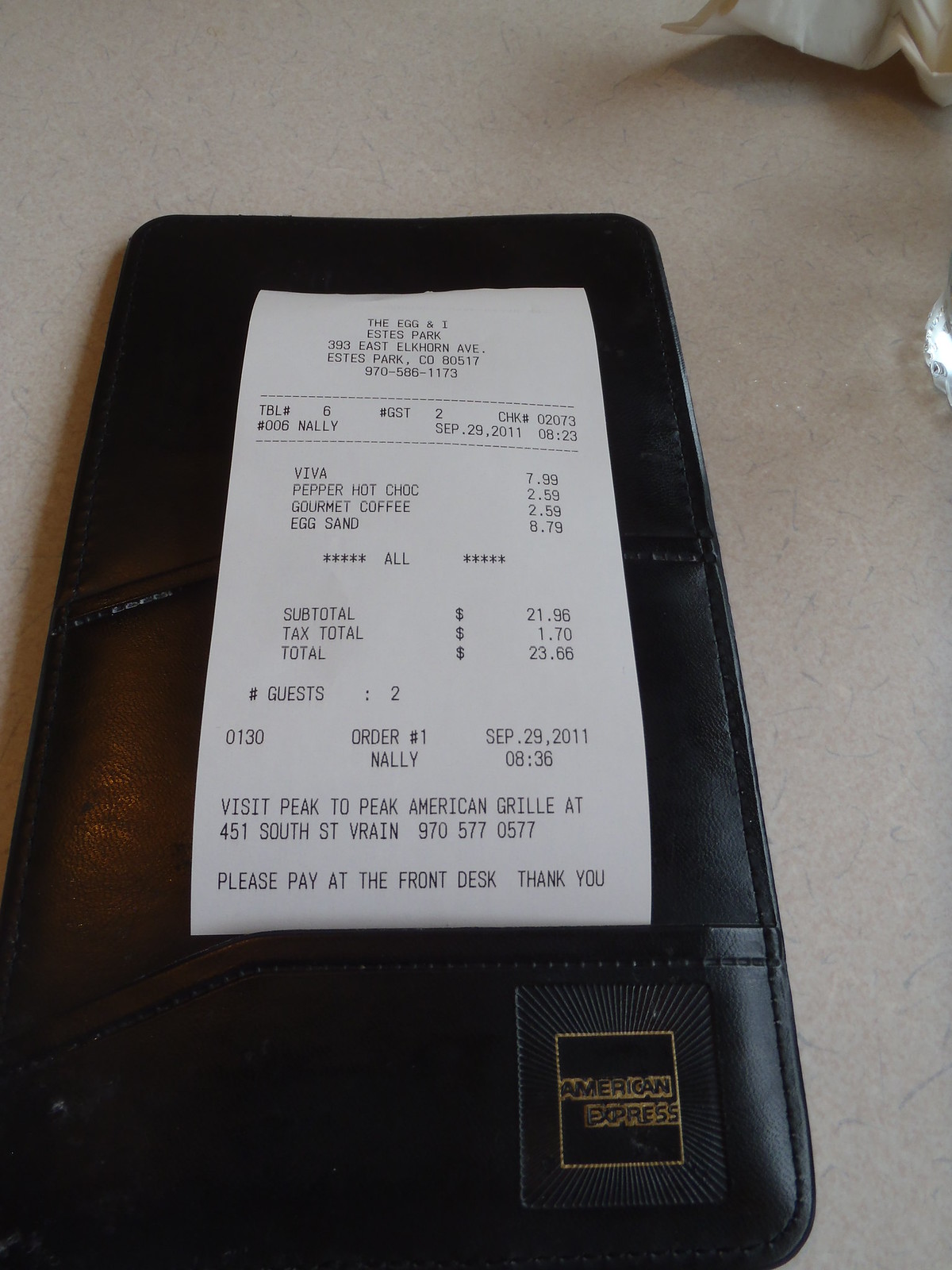This photo captures a restaurant check enclosed in a small black leather case. The case is adorned with "American Express" embossed in gold at the bottom right corner. There's a designated pocket on its exterior for holding a credit card or receipt. Inscribed at the top of the case is "The Egg & I, Estes Park," indicating the restaurant's name and location in Estes Park, Colorado.

The detailed bill outlines an order consisting of a Viva, pepper hot chocolate, gourmet coffee, and egg salad. The total amount, including tax, comes to $23.66. Additionally, the message "Visit Peak to Peak American Grill" is featured, followed by instructions to "Please pay at the front desk. Thank you." The check and its case rest on a light-colored surface, providing a soft contrast to the dark leather.